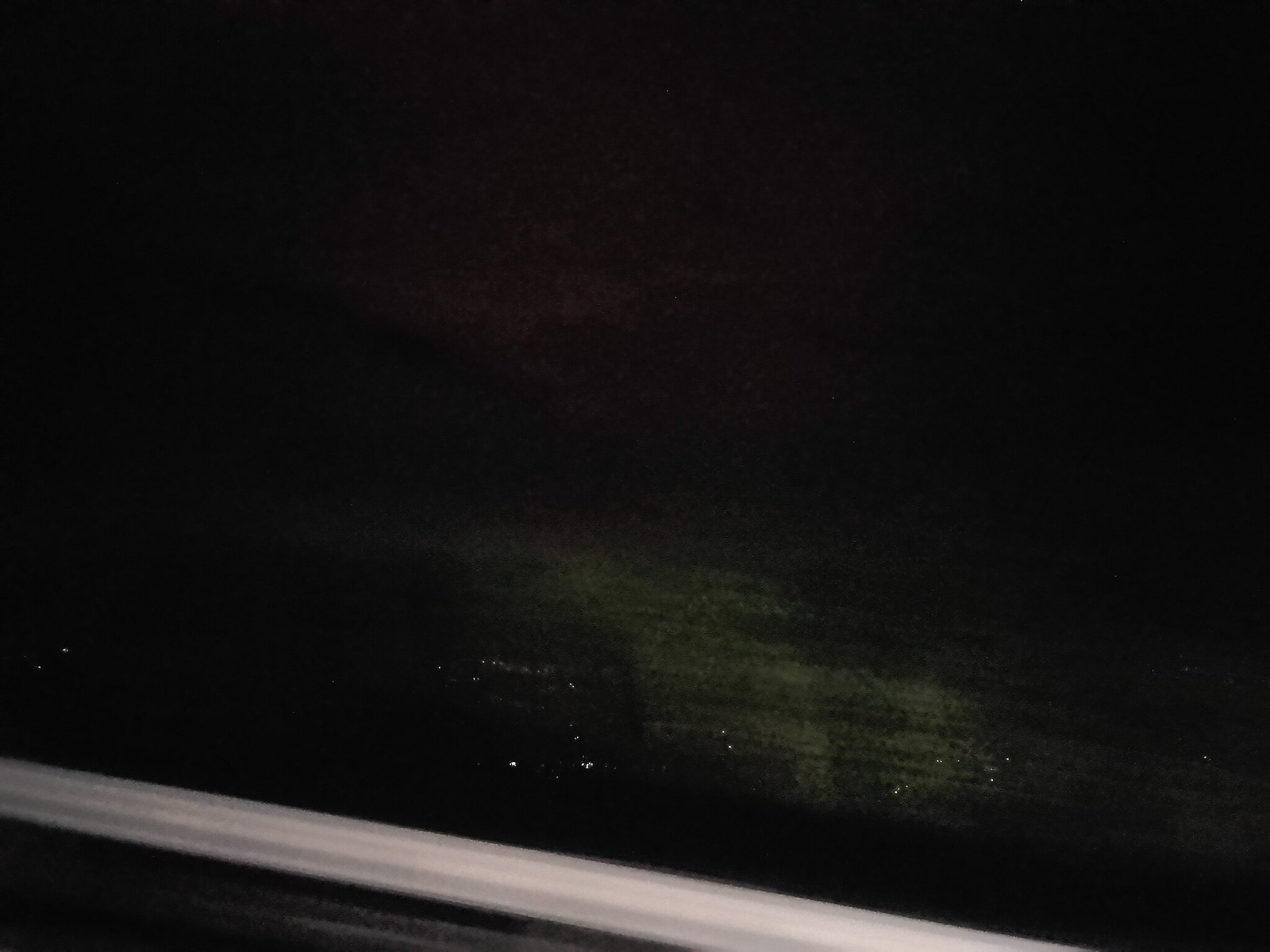The image is predominantly dark, with pitch-black areas dominating the top right, the bottom left, and the left side. In the center of the image, there is a green hue interspersed with brown towards the upper center. A prominent white rail runs horizontally near the bottom, slightly tilting towards the bottom right. Below this white rail exists a darkened counterpart. Scattered across the center and right, with a few on the left, are small white dots, which may suggest distant lights, possibly from a city or industrial site. The overall scene appears to be taken from an elevated perspective, potentially overlooking a body of water, a landscape shrouded in darkness, with faint traces of smoke, giving it an eerie yet intriguing feel.